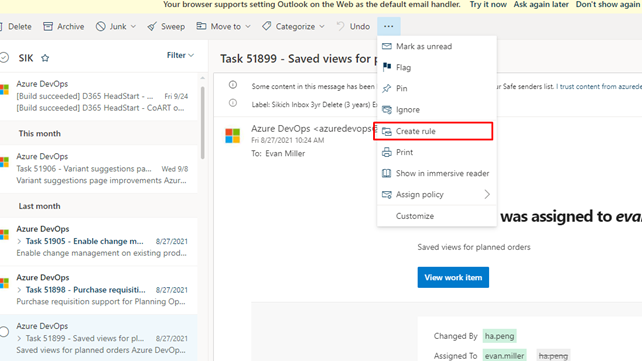At the top of the page, a prominent yellow banner stretches from left to right, informing the user that their browser supports setting Outlook on the web as the default email handler, with options to "Try it now," "Ask again later," or "Don't show again." 

Below the banner, on the left side, there are several gray options listed: "Delete," "Archive," "Junk," "Sweep," "Move to," "Categorize," and "Undo," each accompanied by a small icon. Adjacent to "Undo" on the right, there is a blue square with three dots.

Beneath this section, the text "S-I-K" appears with a small blue star next to it, followed by the word "Filter." Below, it displays "Task 51899, save views for," and a white banner with the options "Mark as unread," "Flag," "Pin," "Ignore," and "Create rule," the latter of which is highlighted with a red marker box. Further options listed include "Print," "Show in immersive reader," "Assign policy," and "Customize."

To the right, there is a partially cut-off note indicating that the task was assigned to "EVA." The text continues with "Save views for planned orders," followed by a blue banner stating "View work item" in white. At the bottom, "Changed by" is followed by a green banner with "H-A dot P-E-N-G" and "Assigned to" is followed by another green banner listing "Evan dot Miller." On the right, a gray banner repeats "H-A ping."

Underneath the "S-I-K" section on the far left, a series of entries labeled "ZURR Develop Ops" are shown, each with additional context. They are categorized by time frames: "This month," "Last month," each followed by tasks and dates. 

Examples include:
- A blue-shaded box mentions "ZURR Develop Ops" with an unchecked circle and "Task 51899, save views for P-L dot dot dot, 08-27-2021, save views for plan orders, ZURR D-E-V op."
- Another task, "51905, enable change M dot dot dot, 08-27-2021," and "Task 151898, purchase requisition 08-27-21, purchase requisition support for planning op."

Each "ZURR Develop Ops" entry is marked with a small square composed of the Google colors: red, green, blue, and gold.